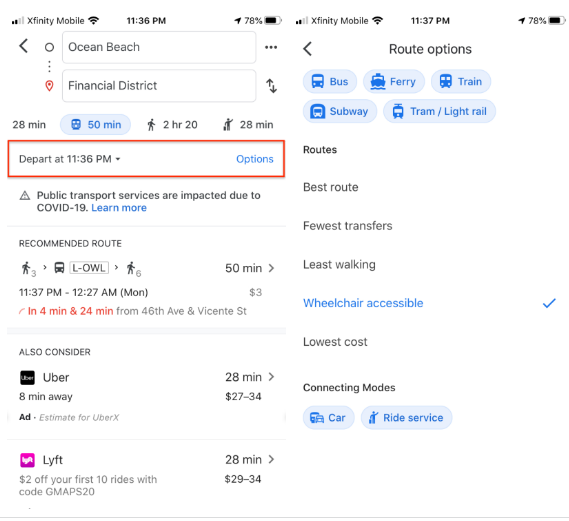In the given image, we observe a website interface related to transportation options. At the top right corner of the interface, a battery icon reveals a charge level of 78%. Adjacent to it, the time is displayed as 11:37 PM, and to its left, there is a Wi-Fi signal strength icon next to the name "Affinity Mobile". In the top left corner, a phone signal strength icon shows two bars.

The image is vertically split into two sections. The right section is titled "Route Options" prominently at the top center. Below this title are five options, each displayed in individual bubble icons. The first bubble on the top left represents a bus with both the word "bus" and an accompanying image. To its right, the second bubble denotes a ferry, followed by a train symbol in the third bubble. The two bottom bubbles indicate subway and tram options, respectively, with corresponding images beside each word.

Below these transportation options, the interface presents various route choices categorized as "Best Route," "Fewest Transfers," "Least Walking," "Wheelchair Accessible," and "Lowest Cost." Notably, the "Wheelchair Accessible" option is highlighted in blue, suggesting it is the selected or recommended route.